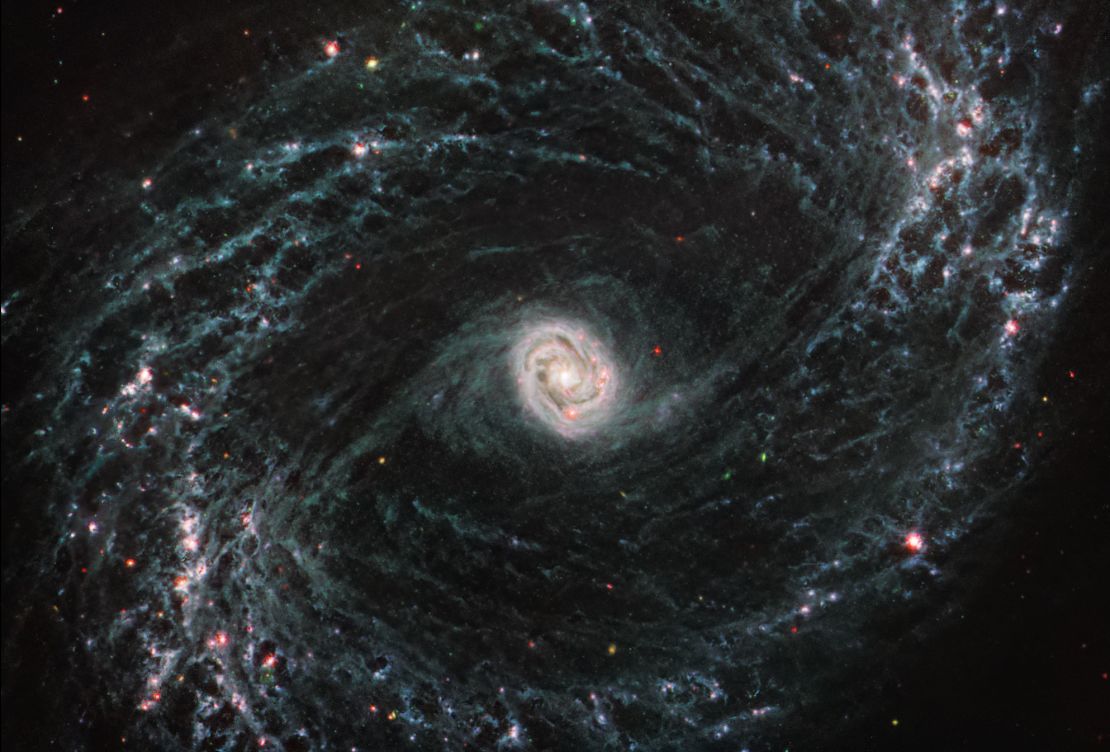This image depicts a possibly old, low-quality photograph of a spiral galaxy in space, taken through a telescope. Set against a plain, pure black background, the galaxy captures the viewer’s eye with its luminous center. At the core, a brilliant white mass, tinged with hints of light pink and brown, likely represents an intensely bright area, possibly a black hole. This central mass is almost white and appears to be sucking in matter, creating a vivid, spiraling effect. Spiraling from this bright core are delicate, bluish-green and white lines forming the galaxy’s arms, which twist elegantly around the center. These arms are punctuated with vibrant white and red spots at their extremities, and the entire image is scattered with white, red, yellow, and green dots, representing stars, nebulae, or other astronomical entities. The concentrated blue and white streams of light emanating from the core, along with the various colored dots, suggest dynamic activity, reminiscent of a star nursery within this awe-inspiring galactic spectacle.